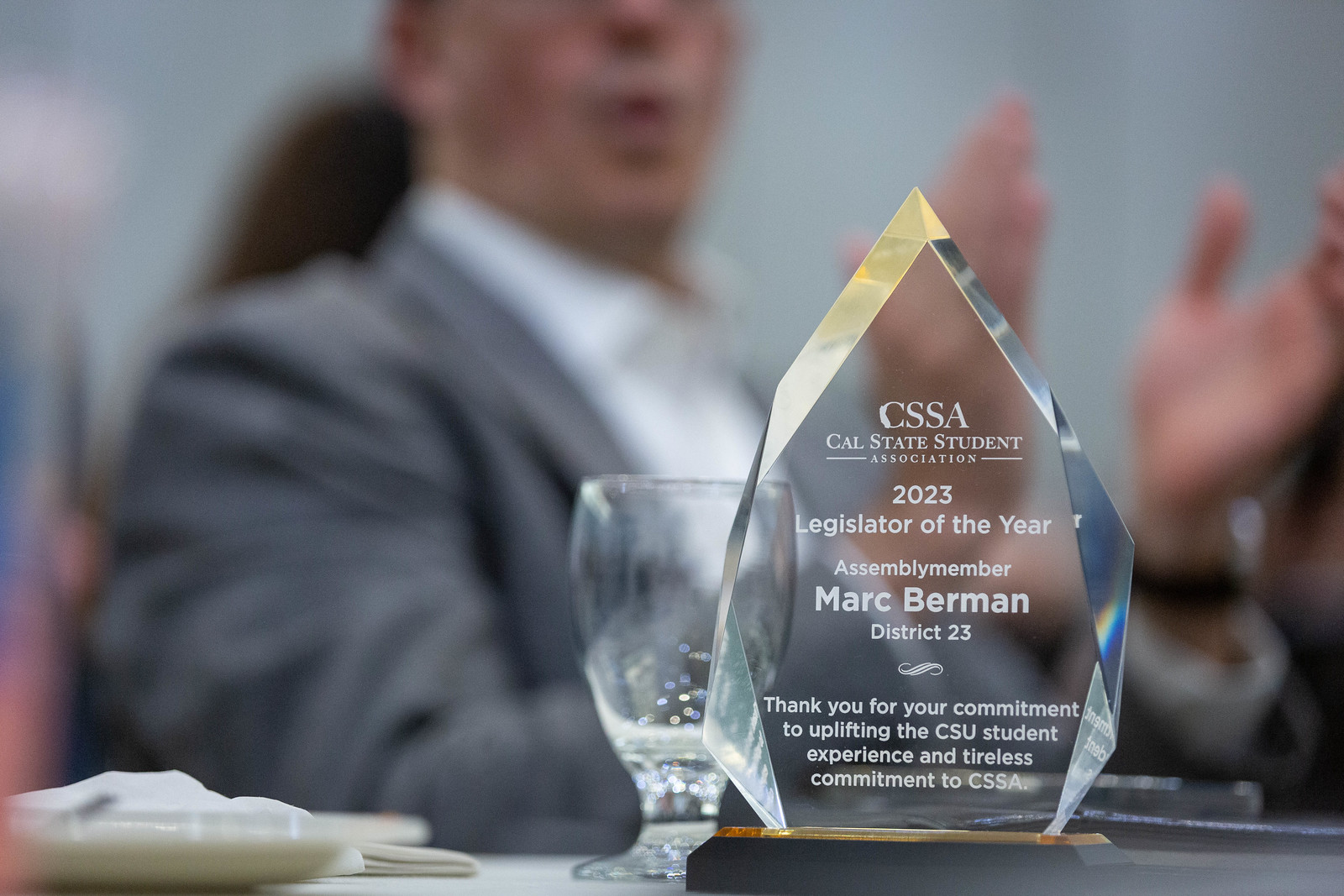The image showcases a close-up of an elegant, upside-down tear-shaped trophy made of clear, cut glass with white inscriptions. At the top of the trophy, it reads "CSSA Cal State Student Association." Below, it honors "2023 Legislator of the Year, Assemblymember Mark Berman, District 23," and includes a note of gratitude: "Thank you for your commitment to uplifting the CSU student experience and tireless commitment to CSSA." Behind the trophy, there is a see-through class, and to the left, a glass is partially visible. In the blurred background, a man wearing a grey suit and a white shirt, with a black watch on his left wrist, is enthusiastically clapping with both hands raised. Along the bottom left corner of the image, there appear to be white items, possibly a cloth napkin and a plate.